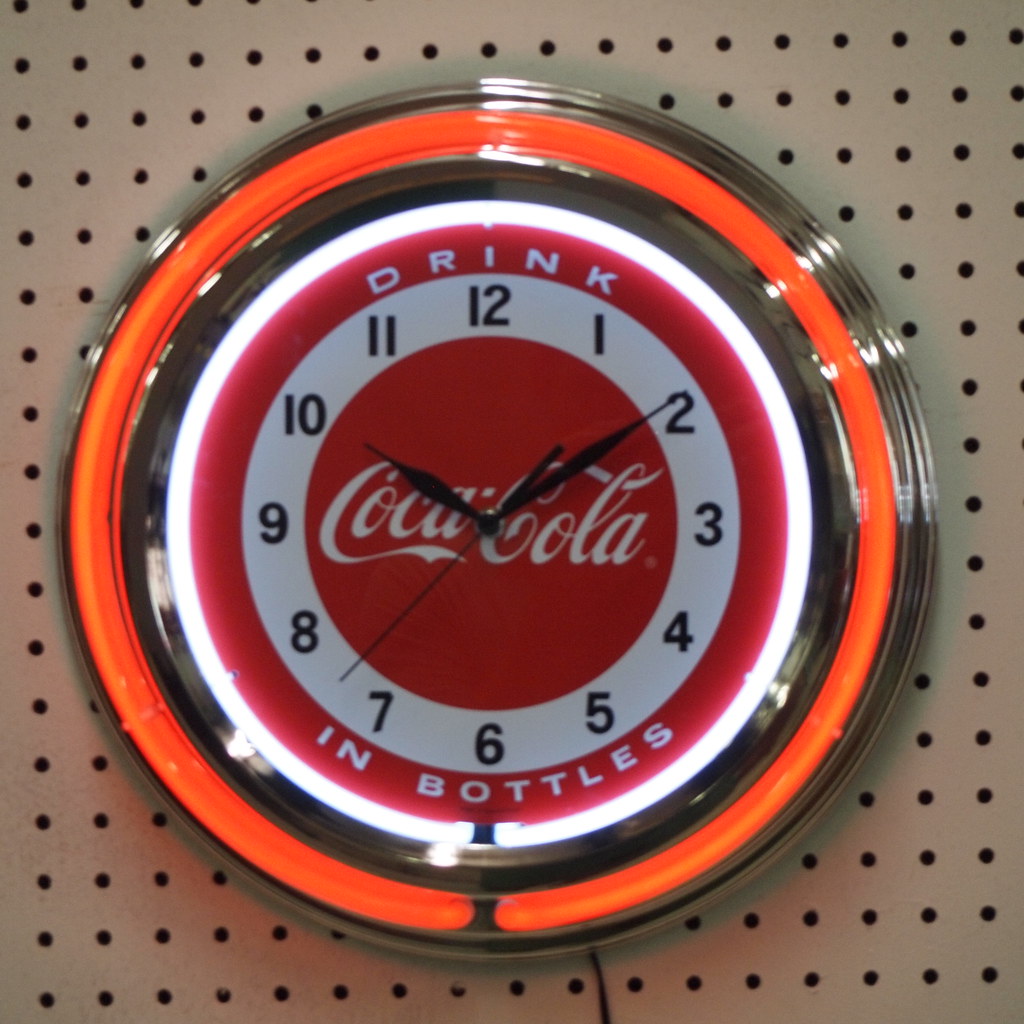This image depicts a Coca-Cola-themed clock prominently displayed on what appears to be a light gray, perforated metal rack commonly found in stores. The clock's outer rim features a gold color, followed by a bright orange border that transitions into another gold circle. Inside this, there is a white-lit circle with markings for the hours and minutes. The most central circle, which catches immediate attention, is a bright red with the classic Coca-Cola logo in white lettering. Positioned at approximately 10:09, the hour and minute hands are also situated within this central red circle. An additional notable feature is the text "Drink" at the top and "in Bottles" at the bottom of one of the inner circles, both written in white on a red background, emphasizing the vintage Coca-Cola branding.